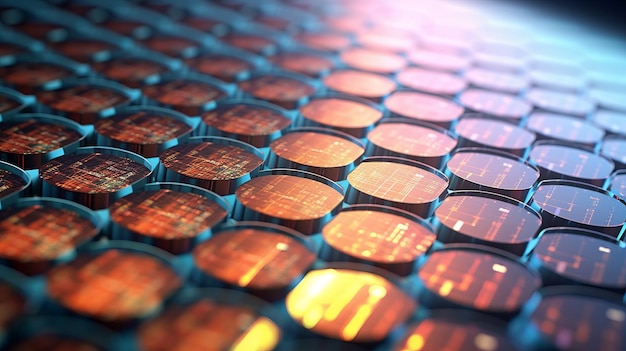This image appears to be a close-up view of a complex set of technological components. Dominating the scene are numerous orange, circular items, which are embedded in a grid-like pattern. These circles vary in brightness, with some exhibiting a glowing, lighted appearance, while others are more muted and matte. The circles also feature fine lines running across them, and each one is surrounded by a raised lip that gives it a distinct shape and texture.

The overall layout of these circles resembles a computer grid, evoking a sense of intricate technology. The background they are set against is predominantly turquoise, adding a contrasting hue to the orange circles. Notably, the top right corner of the image displays a blue halo surrounding the items, which transitions into a black background.

Interestingly, the array of circular items, with their repetitive pattern and varying levels of illumination, also draws a resemblance to microscopic lenses lined up in succession. The image has a certain depth, as the circles near the front of the image are more sharply defined and bright, while those in the background are blurred, creating a sense of movement and focus.

Overall, the image captures the detailed textures and lighting of a technologically advanced grid, possibly resembling computer hardware or a microscopic array.